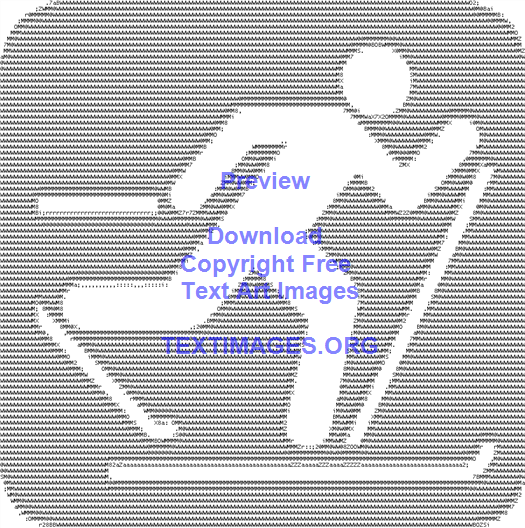In this square image with rounded corners, intricate patterns of black lines, composed of tiny letters and numbers, create an artwork that closely resembles an old Lite-Brite game. At the center, a white stick figure with disproportionately thick body parts is depicted skiing. This figure is artistically carved out by leaving negative space amid the dense rows of characters. The arms of the stick figure are bent at the elbows; one arm extends forward, hold a ski pole that stretches diagonally upwards to the left, while the other arm reaches backward with a ski pole extending horizontally. The legs of the figure show one ski flat on the ground and the other elevated at an angle, both skis curving up at the tips. A blue watermark overlays the image, reading "preview, download, copyright free text, textimages.org." This unique graphic design showcases a creative blend of typographic symbols and computer characters to form a visually engaging piece.